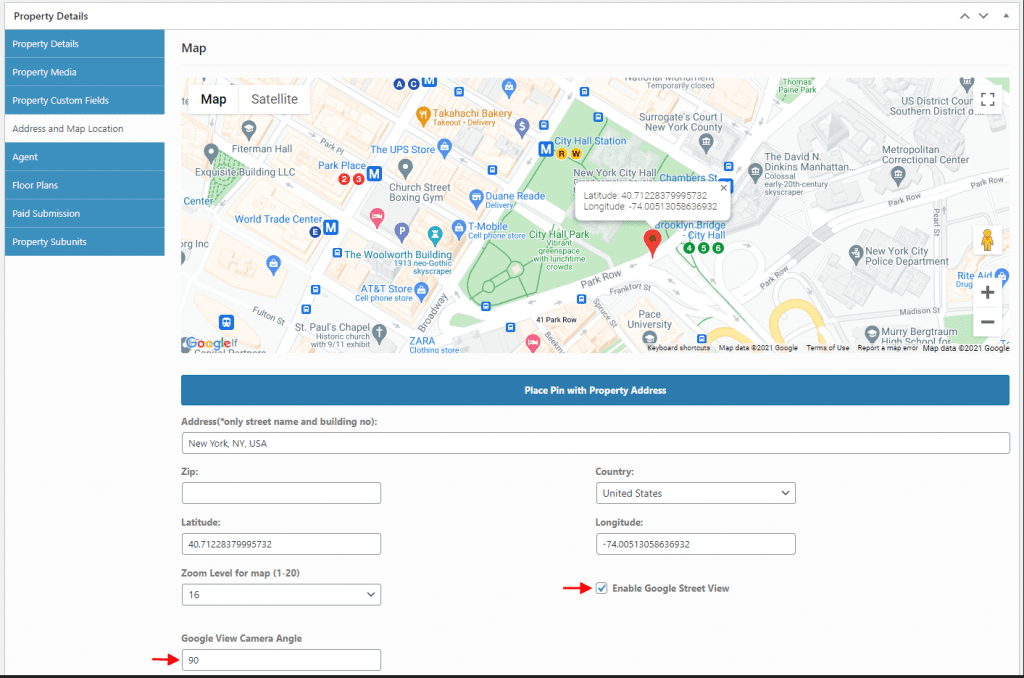**Detailed Caption:**

The image presents a user interface featuring a comprehensive map display layered over a predominantly white background. At the top, a header labeled "Property Details" is prominently displayed. Below this header, there is a horizontal menu bar encompassing several blue square icons. These icons are labeled for navigation and functionality: "Property Details," "Property Media," "Property Custom Facts," "Adjusts," and "Floor Plans."

To the right of these elements resides a detailed map of New York City. The map allows for toggling between "Map" and "Satellite" views, indicated at the top. The map showcases numerous landmarks and public places marked with various colored markers: blue and red, predominately. Key landmarks such as the New York City Police Department, World Trade Center, AT&T Store, St. Paul's Chapel, a gym, a bakery, and expressive greenery suggesting a park are illustrated. However, it is unclear if this green space is Central Park as it is not explicitly indicated.

Adjacent to the map, a side panel features various controls and fields: a search bar pre-filled with "New York, New York, USA," an empty ZIP code field, latitude coordinates, zoom level (preset at 16), Google View Camera Angle (set at 90 degrees), longitude code, and a drop-down for specifying the country (set to United States). The bottom-most option in this panel offers an ability to enable Google Street View. These settings suggest customizable map navigation and detailed property pinpointing capabilities.

To the far right of the image, typical navigational icons are present, including a person icon and a golden map marker. The design and functions depicted suggest a robust tool or application for real estate management or spatial analysis in New York City.